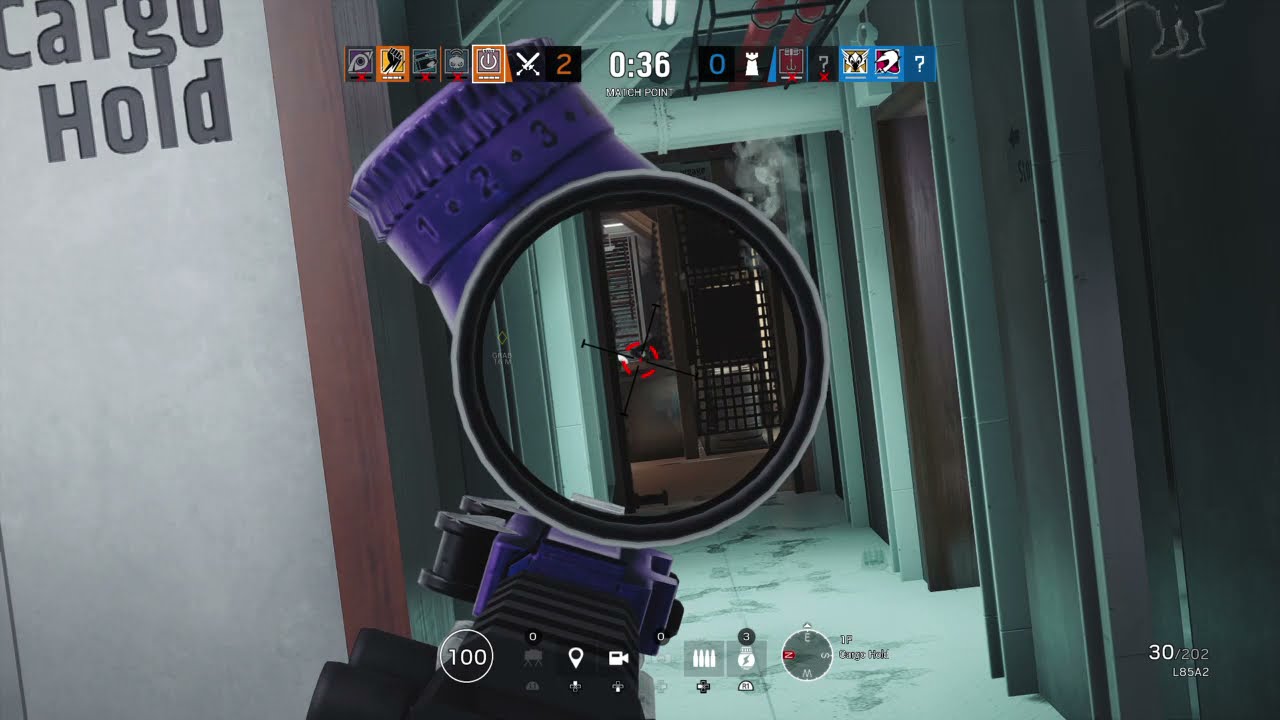In this detailed screenshot from a first-person shooter video game, a black and purple gun with an attached scope is centrally positioned, aiming into the background where a long corridor or hallway extends forward. The corridor features green flooring and green door frames, with walls of copper, white, and brown tones. At the top left of the screen, gray text reads "cargo hold," while in the top middle, a banner displays multiple game emblems, suggesting a competitive match. The center of the screen prominently displays the text "match point." The bottom right corner of the image displays the numbers "30/202 laser," and additional numerous symbols and numbers are scattered across the screen. The overall aesthetic, combined with no visible characters, emphasizes the scene’s focus on combat or tactical gameplay, underlined by the targeting mechanism locked onto a wall further down the hallway.